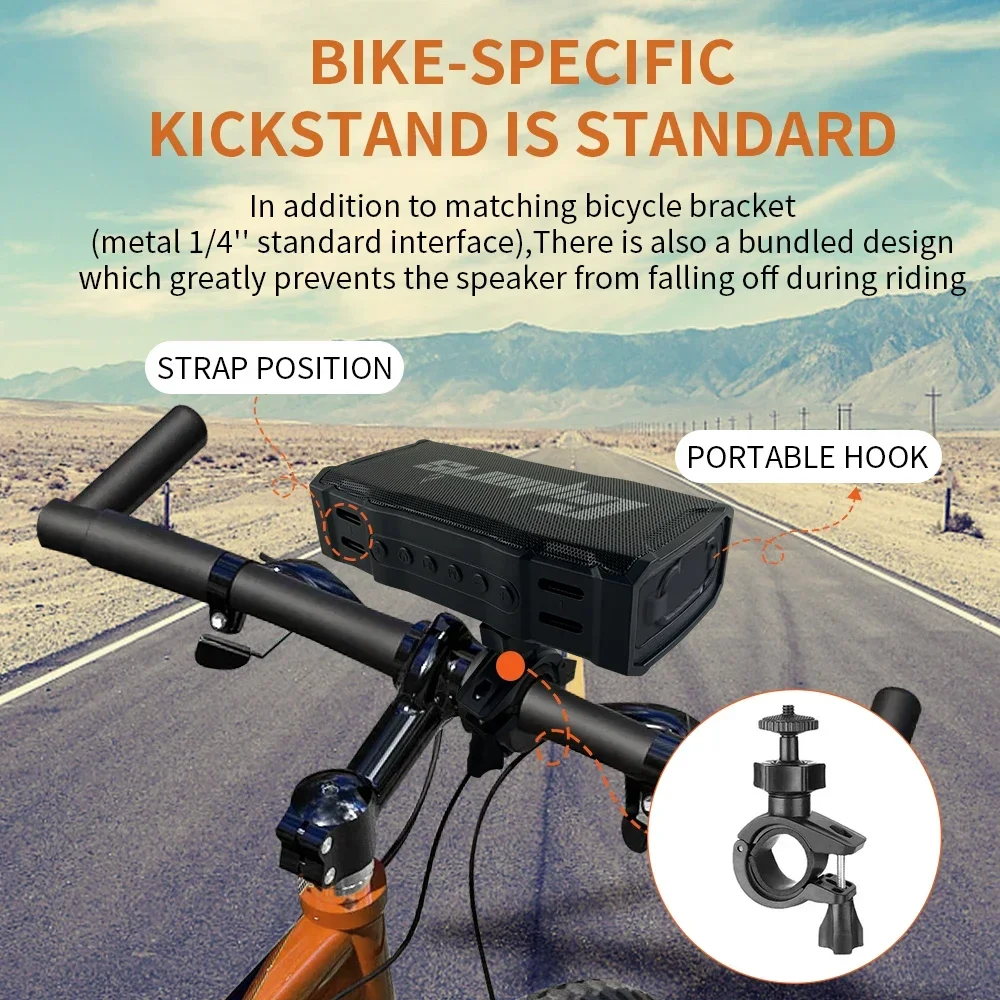This advertisement features a striking square photograph of a desert highway scene. The mid-afternoon haze adds an ethereal quality to the backdrop, where a two-lane blacktop road stretches into the distance towards a mountain ridge. Telephone poles line the road, flanked by patches of brown desert sand and sparse vegetation.

In the foreground, the handlebars of a bicycle take up the bottom half of the advertisement. Mounted on the handlebars is a black speaker adorned with numerous buttons and a side handle. The speaker's securing mechanism is highlighted, with an inset picture at the bottom right showing a close-up of the circular clamp and its round knob. Labels on the speaker detail its features, with "Strap Position" marked on the left and "Portable Hook" on the right, both in black writing on a white background.

A beige headline at the top reads, "Bike-Specific Kickstand is Standard." Below, additional black text states, "In addition to matching bicycle bracket; metal one-quarter inch standard interface, there is also a bundled design which greatly prevents the speaker from falling off during riding."